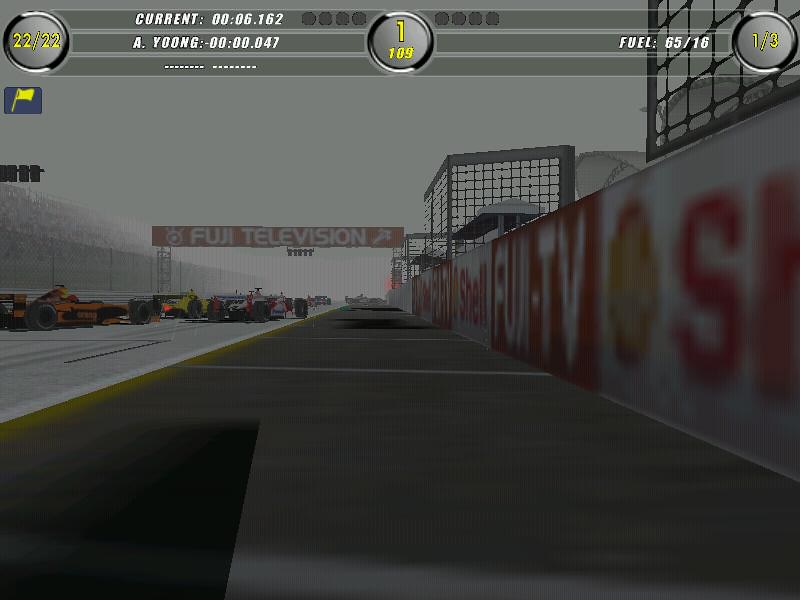The image is a detailed screenshot from a car racing video game, depicting a foggy day at the starting grid. The viewpoint is from the pit lane looking towards the back of stationary cars on the grid, preparing for the start of a race. At least four cars are visible in the foreground, including an orange one, a yellow one, and a multicolored white and red car. The grandstands are faintly visible behind the cars, filled with fans. Overhead, there is a red and white banner displaying "Fuji Television" along with traffic lights hanging down, which the cars will pass under once the race begins. On the right side of the image, advertising banners for Fuji TV and Shell are seen along the wall beside the track, but they appear blurry due to the fog. The top of the screen is filled with various game statistics, including race times, positions, and fuel levels. Specifically, it shows "22:22" in the top left corner, "1 out of 3" in the top right, and the current timing details such as "06:00.162" for the player named "A. Jung," with a comparative time of "-00:00.047". Additionally, the fuel level is indicated as "65%".